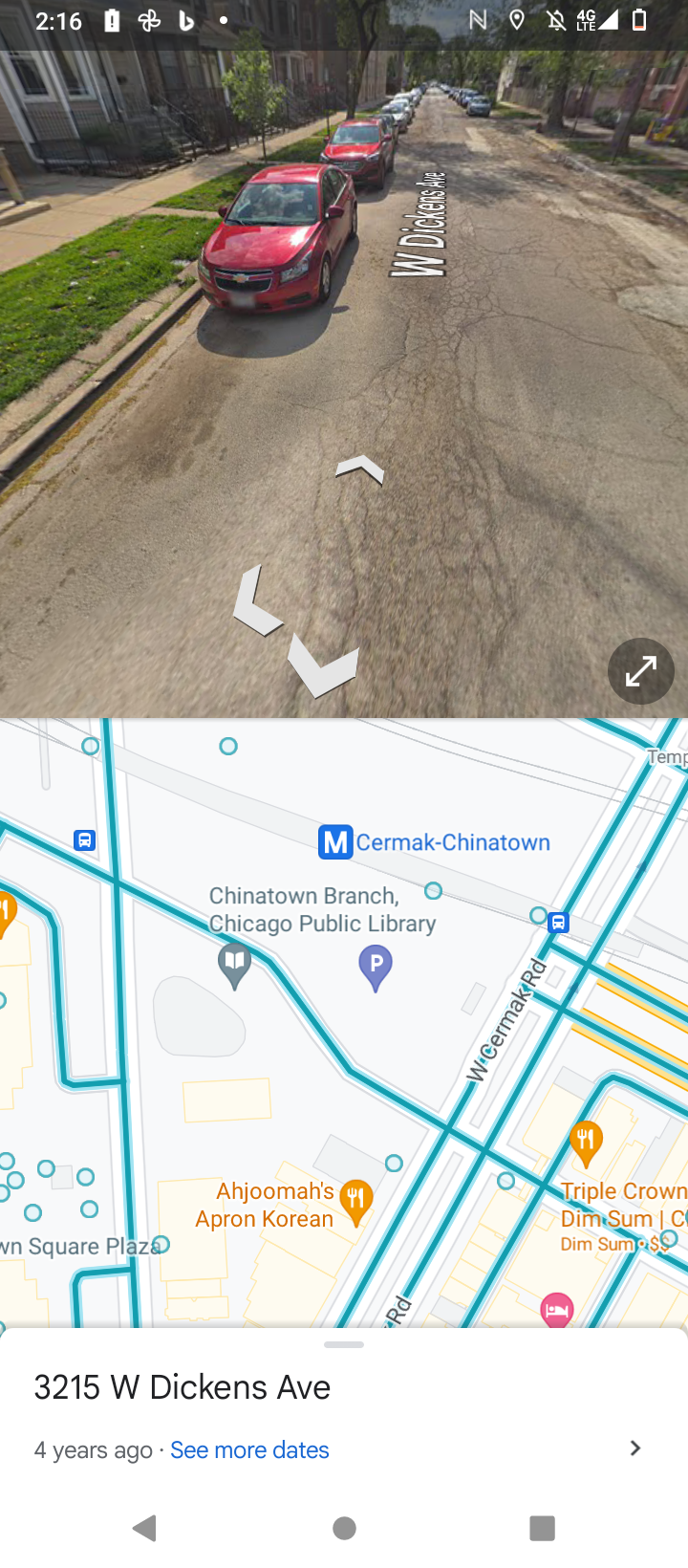The composite image consists of two square images stacked vertically. The top image depicts a brown street, labeled "West Dickens" in white letters that diminish in size towards the background. Two red cars are parked facing the viewer's direction on the street, which is flanked by a sidewalk and patches of grass to the left. Partially visible buildings line the edge of the street beyond the sidewalk.

The lower image is a map, resembling a Google map, with an address "3215 West Dickens Avenue" written in black text below it. A timestamp indicating "four years ago" is written beneath the address, followed by the name "Seymour Gates" in blue text. The map features blue lines representing the streets against a white background, interspersed with pale yellow sections and variously colored markers, including purple, red, and orange. The street layout shows one vertical street running from the top left to the lower right while two streets extend from the upper right corner towards the lower middle. Various other streets are also depicted.